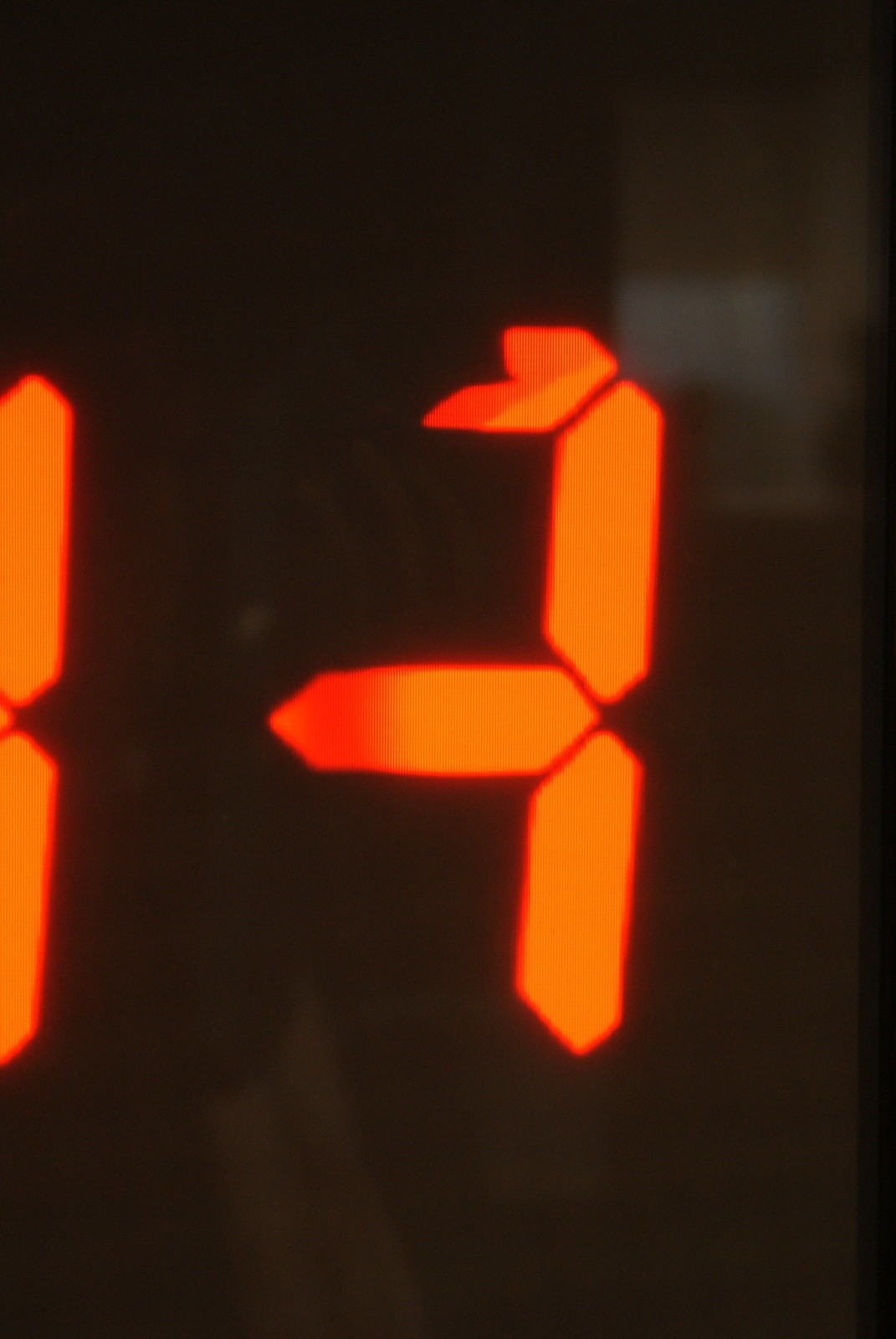Up-close photograph of a malfunctioning LED display. The right side of the image features one vertical bar at the top, followed by another vertical bar below it, and a jagged, partially illuminated horizontal bar intersecting the middle section. The top left area of the supposed horizontal bar is incomplete and irregular, indicating a malfunction. The absence of a crucial bar at the bottom leaves the representation unrecognizable as any specific number. Additionally, two vertical bars on the far left hint at the presence of another number on an adjacent display.